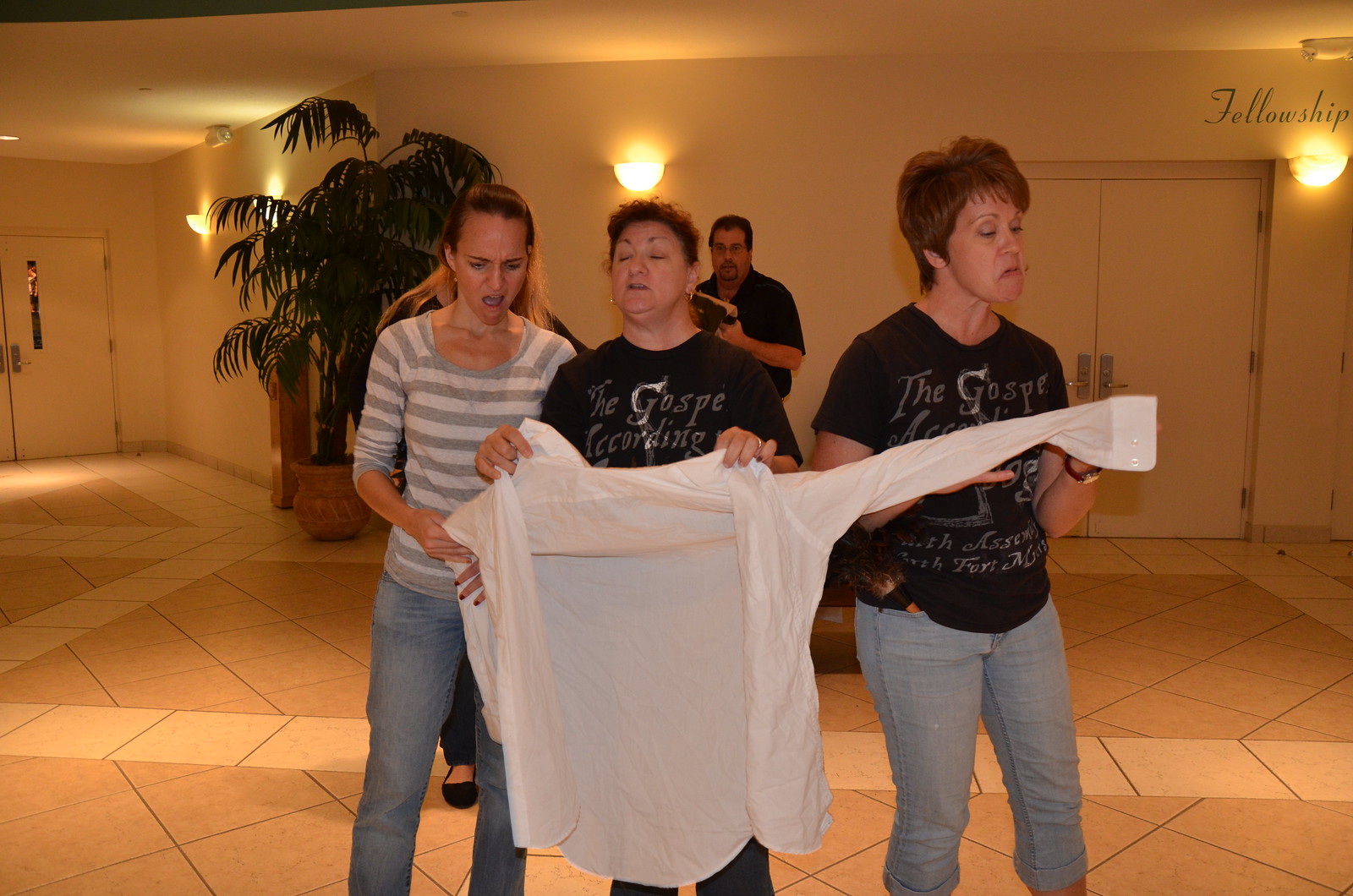In this detailed indoor scene, three women stand shoulder-to-shoulder as they hold a white long-sleeve button-up shirt. The woman on the left is younger and wears a white and brown-striped t-shirt paired with jeans, with a somewhat disgusted expression. The woman in the middle dons a black t-shirt with gray lettering that reads "The Gospel Recording," and similarly wears jeans. The third woman, on the right, also sports a black t-shirt with the same lettering, and appears slightly annoyed as she grasps the sleeve of the shirt. All three face the camera, capturing a moment of candid interaction. Behind them, a man stands by a white wall, seemingly entertained by the scene. The room features several lights on the wall, a palm tree to the left, and two sets of double doors—one to the far left and another visible on the right side of the image. The floor consists of square tan tiles, and the word "Fellowship" is visible on the wall in the upper right corner.